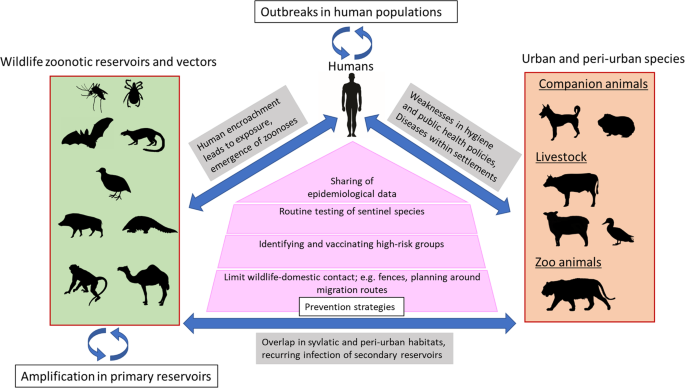The image presents a detailed chart outlining the dynamics of zoonotic disease outbreaks among human populations. Central to the illustration is a rectangle at the top labeled "Outbreaks in Human Populations," with a human figure beneath it. Double-sided arrows extend from this figure, emphasizing interactions with various elements. 

On the left, a green rectangle titled "Wildlife: Zoonotic Reservoirs and Vectors" contains silhouettes of various wild animals. Opposite on the right, a pink rectangle labeled "Urban and Peri-Urban Species" features icons of companion animals, livestock (such as cows, sheep, and ducks), and zoo animals (including a tiger). These sections highlight the different sources of zoonotic transmission.

Intricate double-sided arrows circulate around these primary elements, with some specifically noting "Amplification in Primary Reservoirs" and "Overlap in Sylvatic and Peri-Urban Habitats Regarding Infection of Secondary Reservoirs." 

Additional annotations include "Human Encroachment Leads to Exposure and Emergence of Zoonosis" on the left side and "Weaknesses in Hygiene and Public Health Policies, Diseases Within Settlements" on the right. Lower down, a pink triangle advises "Sharing of Epidemiological Data, Routine Testing of Sentinel Species, Identifying and Vaccinating High-Risk Groups," and suggests the need to "Limit Wildlife-Domestic Interaction."

This chart aims to elucidate the various factors influencing zoonotic disease outbreaks, emphasizing interspecies interactions and preventive measures.